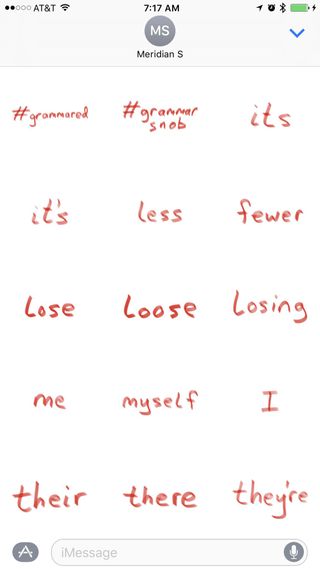This image is a screenshot taken from someone's cell phone, specifically from an iMessage conversation. The recipient's name, "Meridian," is displayed at the top of the screen, alongside the cell phone network details, indicating that the phone is connected to Wi-Fi, the battery is fully charged, location services are active, an alarm is set, and Bluetooth is enabled. 

Unconventionally, the main portion of the screen deviates from the typical iMessage format of alternating speech bubbles. Instead, it features what appears to be a handwritten graphic, filling the entire screen with three columns and five rows of text. The handwritten notes are categorized in a structured, grid-like format. The content includes grammatical corrections and distinctions between commonly confused terms such as "its" versus "it's," "less" versus "fewer," "lose" versus "loose" and "losing," "me" versus "myself" versus "I," and the various forms of "their" ("their" as in possession, "there" as in location, and "they're" as in they are). The hashtag "#grammarsnob" is positioned at the top of this handwritten list, indicating a focus on grammatical accuracy.

The bottom of the screen confirms the use of iMessage, showcasing the unique and organized manner in which the sender has communicated these grammatical points, likely as part of a personalized or educational message.